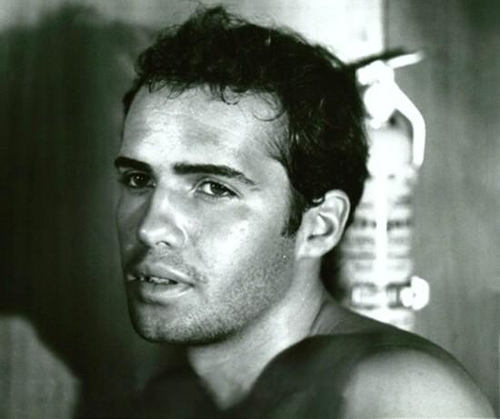This black-and-white photograph features a striking, shirtless young man, who might be the famous Marlon Brando in his early 20s. The subject has dark, curly hair that appears wet, possibly from engaging in a vigorous activity such as boxing. He sports a five o'clock shadow and dark eyebrows, enhancing his conventionally attractive and calm presence. The man gazes into the distance with a slightly open mouth, exuding a sense of collected composure. In the background, a gray wall with lighting casts a shadow of his head. A silver object resembling a fire extinguisher is mounted on a pole behind him, adding an intriguing element to the scene. The image captures the subject from mid-shoulders upwards, emphasizing his youthful vigor and intense expression.